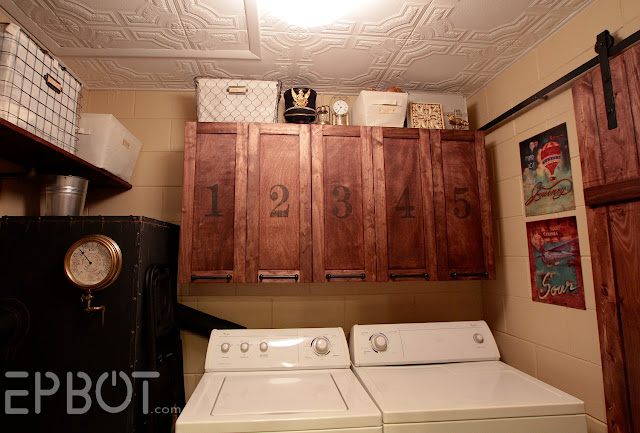The photograph captures a compact laundry room with cement block walls and a tiled ceiling featuring a central light source. Dominating the room are an older style, white top-loading washing machine and a front-loading dryer, side by side, slightly off-center in the frame. Above these appliances, a series of wooden cabinets, numbered 1 through 5 in slightly faded black text with handles on the bottom of each door, provide storage and draw focus. Adding a decorative touch, cloth bins and miscellaneous items rest on top of the cabinets. To the left of the washer and dryer stands an old black water heater or boiler with a bucket placed on it. Adjacent to the appliances, there's a dark brown, old-fashioned trunk with a metal dial resembling a clock. A set of posters, possibly depicting balloons, adorns the wall to the right. The room is completed with a sliding barn door on a bracket.